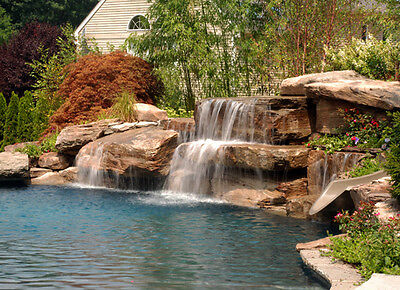This image captures a professionally landscaped residential scene, likely located in a gated neighborhood or upscale community. The focal point is a beautifully designed pond with greenish-blue water that reflects shades of brown and green from its surroundings. This pond is fed by a waterfall that cascades down two different rock formations, adding a dynamic element to the scene. Flanking the pond is additional rock work, and a hidden slide emerges discreetly into the water, adding a playful touch.

The background features a tan-colored building—either a house or a possibly a small church—that appears slightly worn or dirty. An old window is visible at the top of this structure. Half of this building is obscured by a large tree, enhancing the natural feel of the setting. Further into the background, a mix of green and orange foliage enriches the scenery. The image is photographed slightly from an angle rather than straight on, contributing to the professional quality of the photograph likely intended for a company website. The scene is a blend of natural charm and meticulous landscaping, creating an inviting outdoor space.